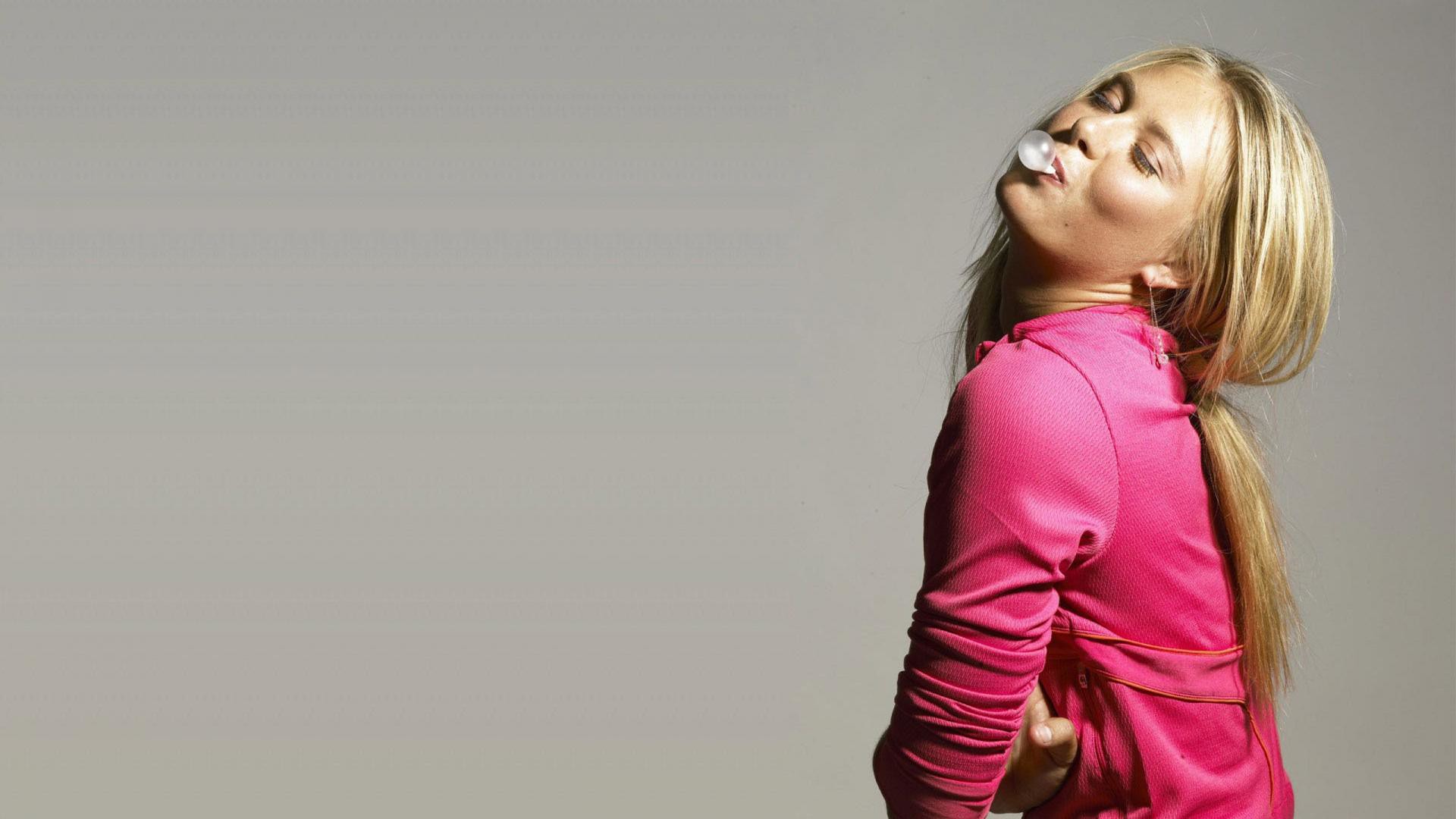The image features a young blonde woman, positioned to the right of the frame, against a taupe background with faded horizontal lines on the left two-thirds. She is wearing a pink long-sleeve top, detailed with a strap around the center. The woman stands in left side profile, her left shoulder facing the camera. Her head is tilted back, face turned towards us, and eyes closed as she blows a white bubble of gum. Her hair is tied back in a loose, slightly messy ponytail, with strands escaping. Notably, she has pronounced cheekbones, suggesting facial fillers, and signs of Botox on her forehead. The woman’s right hand is tucked behind her left arm, which is slightly obscured by the pose. She wears a dangling earring in her right ear, featuring a design of three pearls topped off with a small white ball at the bottom.